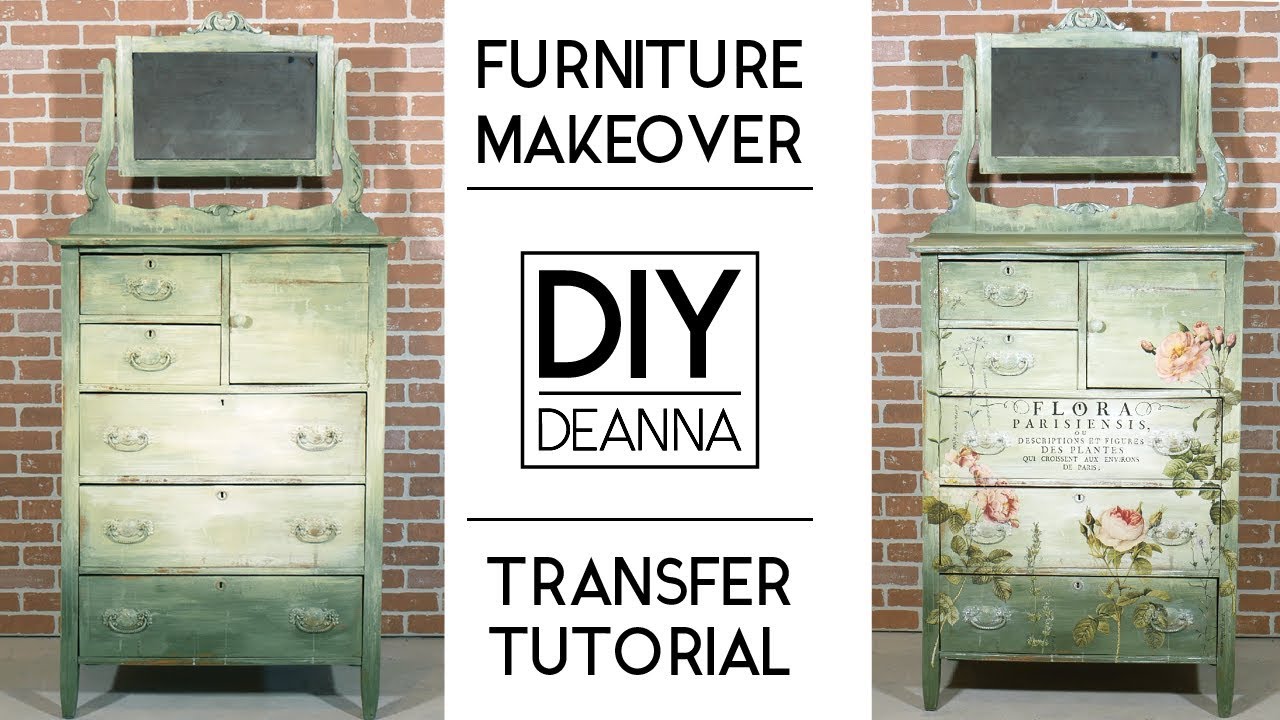The advertisement showcases a DIY Furniture Makeover by Deanna, featuring a Transfer Tutorial. It prominently displays two mirrored images of antique dressers set against a stark black-and-white, brick wall background. The dresser on the left appears plain and worn, characterized by a faded, old-timey shabby chic look in shades of gray and green. In contrast, the dresser on the right has been artistically transformed with vibrant pink flowers and lush green leaves, illustrating the application of floral and text art. The text on the image, "Furniture Makeover, DIY, Deanna, Transfer Tutorial," is central and emphasized in black and white. The visual contrast highlights the transformative potential of adding detailed designs to rejuvenate vintage furniture.